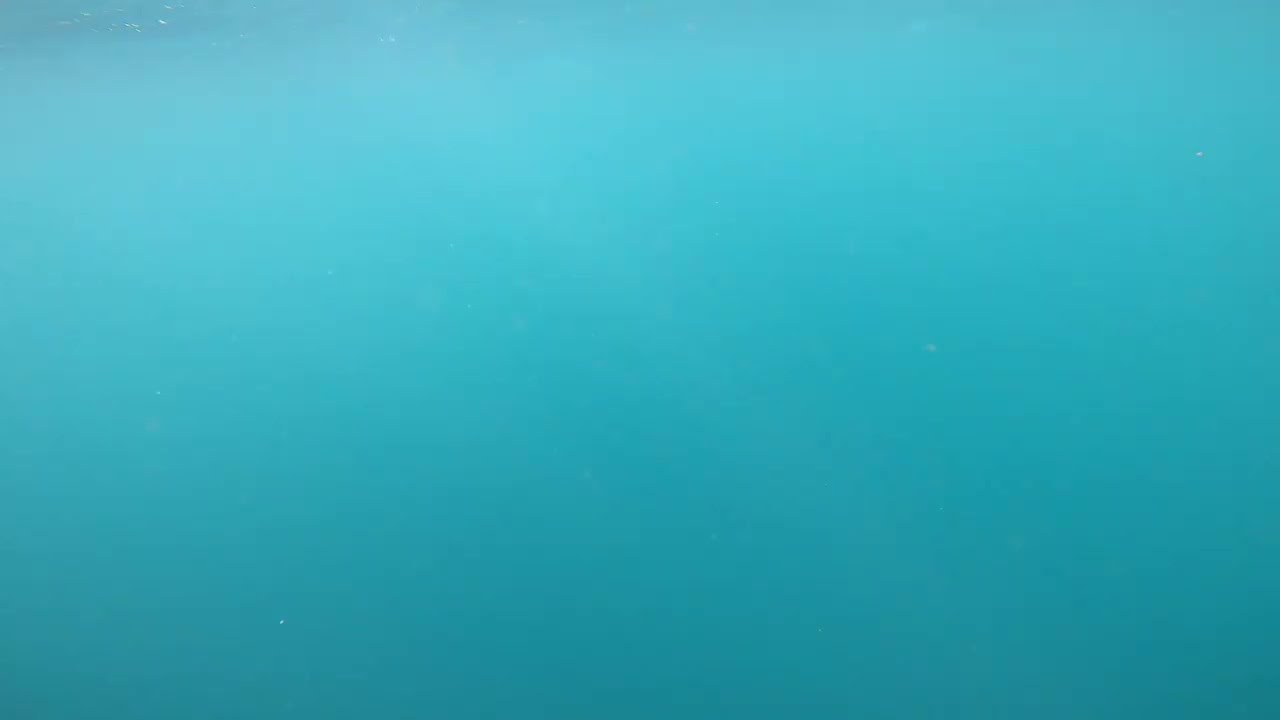This image is a rectangular photograph, longer in length than in width, dominated by a serene blue color reminiscent of a tropical ocean or the sky. The blue shade is lighter in the center, transitioning to slightly darker tones at the top left and bottom right corners. Scattered within the blue expanse, there are a few shining silver dots, most notably in the top left corner and sparingly in other parts of the image. Despite these minute details, the overall impression is of a nearly uniform, tranquil blue landscape.